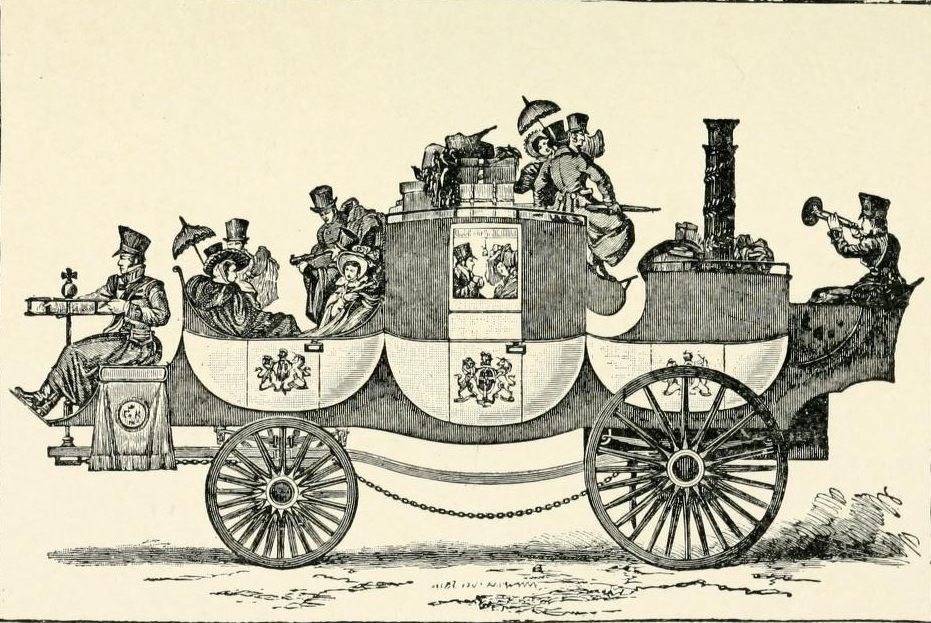This black-and-white drawing features an elaborate, old-fashioned carriage traversing from right to left across a plain cream-colored background. At the forefront of the scene is a man donning a top hat and long coat, seated on a small, striped black-and-white wooden platform. He appears to be steering the vehicle using a horizontally positioned wheel, which is affixed with a round ball topped by a cross. The large stagecoach he commands seems to be propelled by an unseen mechanism, potentially steam, as there are no horses in sight.

The carriage comprises multiple connected compartments. Directly behind the driver section is an open coach area populated by passengers—men, women, and children—all dressed in typical late 1800s attire, including tall hats and heavy coats. Another compartment further back is enclosed, featuring a detailed crest on its doors. Passengers inside this section include a man in a top hat facing right and a woman in a grayish dress facing left. Atop this compartment is a pile of luggage and additional seating, occupied by a man in a gray coat with his back to the viewer and a woman with a parasol barely visible over his shoulder. Another man in a top hat is also seated near the luggage, looking back towards the scene.

The rear section of the carriage houses a conspicuous chimney stack, possibly indicating the vehicle's engine. A man seated here in a conductor’s hat and black shirt appears to be blowing a bugle. The carriage’s unique design includes a large rear wheel and a smaller front wheel, connected by a chain. This intricate and bustling scene reflects the transportation style and social nuance of the late 19th century, brought to life in meticulous black and white detail against a subtle cream background.